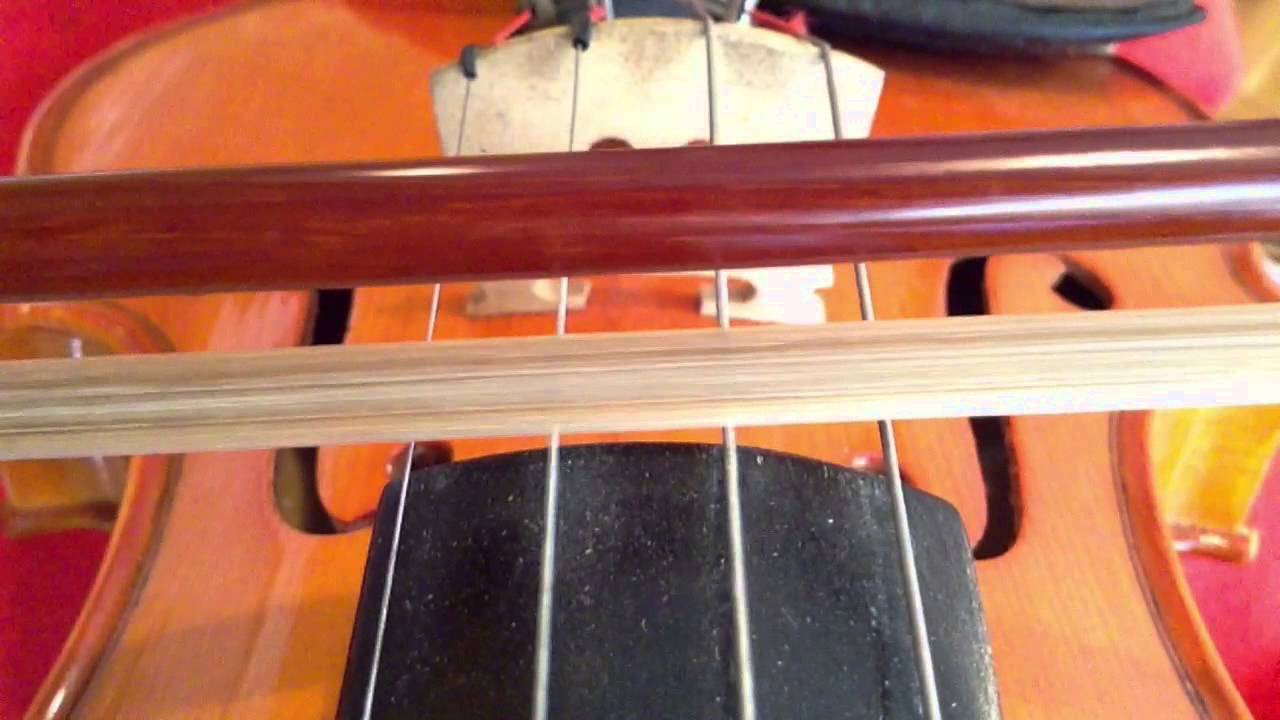This detailed horizontal image captures a close-up view of a beautifully crafted violin. The focal point is on the four meticulously arranged strings that span the length of the instrument, highlighting the fine craftsmanship and precision involved in its creation. Visible cuts in the wood on the violin's body add to the richness and intricacy of the design, showcasing the traditional F-holes that contribute to its resonant sound.

Horizontally positioned across the strings is the bow, with its elegant brown wooden upper frame and white horsehair at the bottom, ready to draw out melodies. The violin rests gracefully on a vibrant red surface, which contrasts with its polished, yellowish-brown sides and ridges, enhancing the visual appeal. A black element, possibly a hand or part of an accessory, is discernible at the top, adding a hint of human interaction with this timeless musical instrument.